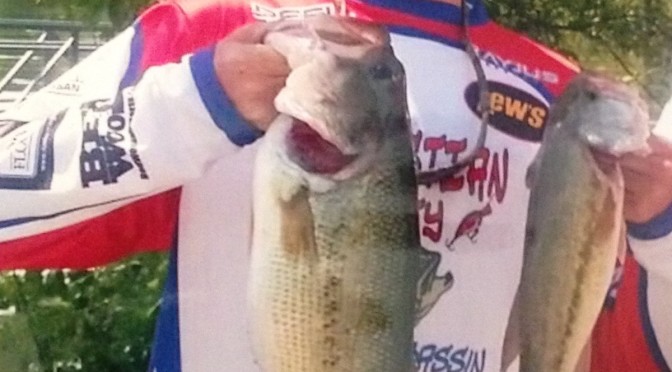In the image, a faceless man is prominently featured holding up two large, pale fish, one in each hand. The cropping of the photograph focuses closely on his upper body, his arms, and the fish, which appear to be about the size of his torso. The man is adorned in a distinctive, multicolored shirt that predominantly features red, blue, white, black, and yellow hues, resembling a racing uniform or possibly fish monger attire. The shirt has blue bands around the sleeves and neck, and a red panel below the neck band and on the arms, adding to its vibrant appearance. The faint text and unclear logos on the shirt suggest sponsorship, with visible letters in yellow reading "E, W," followed by a comma, and then an "S." The setting of the image is outdoors, characterized by lush green vegetation in the background, and a structure that appears to be bleacher seating on the far left. Overall, the picture captures the essence of an enthusiastic fisherman or fish vendor proudly displaying his catch.